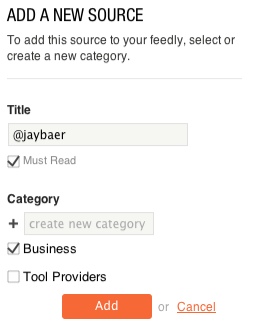The image depicts an interface with a clean, all-white background. In the top left corner, there are bold, all-capital letters indicating a section title. Below this title, in smaller black letters, it reads: "To add this source to your Feedly, select or create a new category." A thin gray line spans horizontally across the image from left to right, providing a visual separator.

Following the line, there is a slight space below it. The text "TITLE" is displayed in bold black letters. Beneath this, a rectangle contains the handle '@jbayer' in black. Below the rectangle, there is a square with a black checkmark inside, and to its right, the text "MUST READ" is written in gray.

Moving further down, there is another bold black label "CATEGORY." Underneath this, a black plus sign is situated to the left of a gray rectangle containing the text "Create New Category." Continuing down the left side, there's a square with a black checkmark next to the word "BUSINESS" in black text. Below this, there is a white box outlined in black, with the text "Pool Providers" to its right. An orange tab labeled "ADD" in white is located under the 'R' in "Providers." To the right of this tab, the word "or" appears in small grayish text.

In the bottom right corner of the image, the word "CANCEL" is seen in red, underlined with a red line, finalizing the interface details.